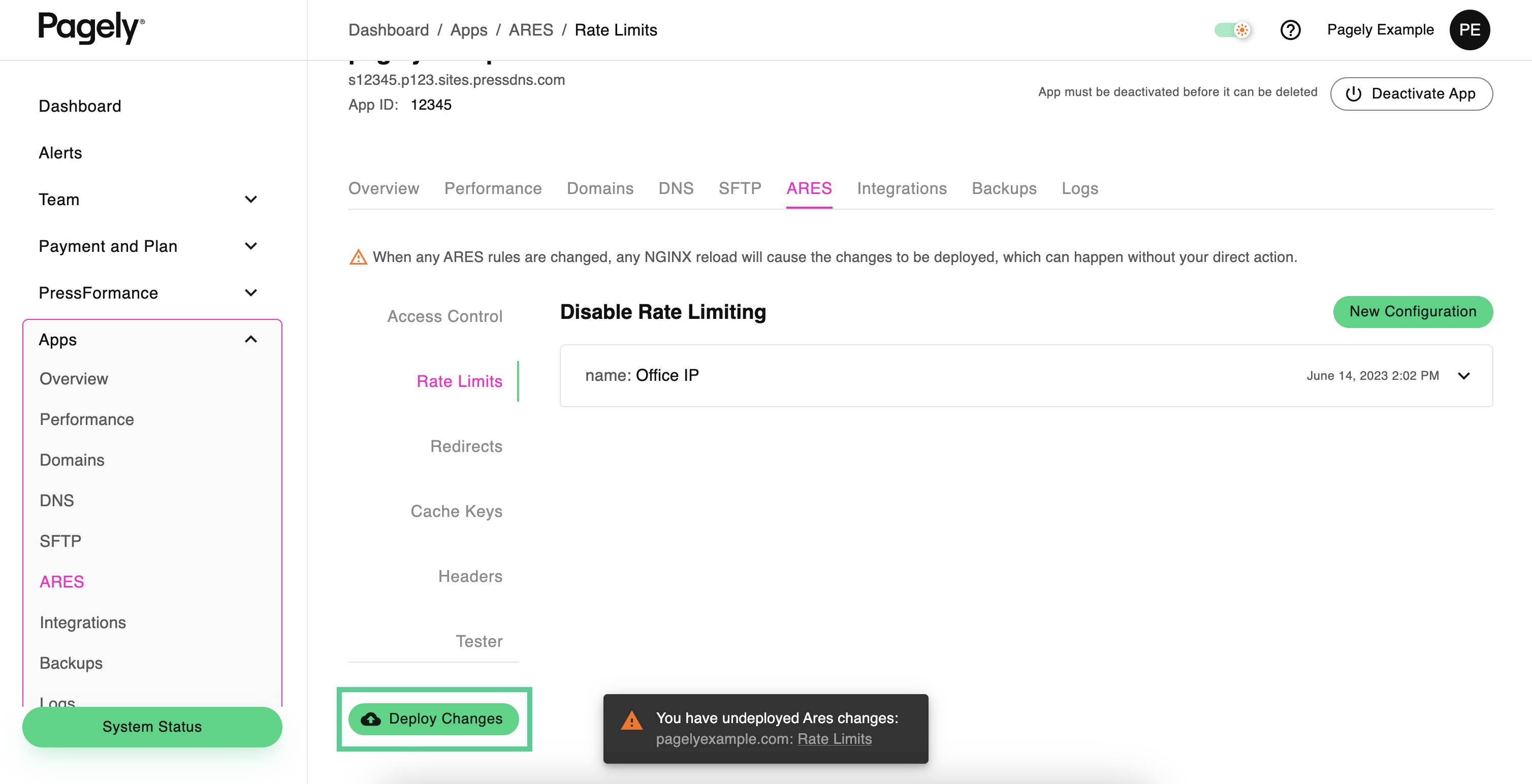The image depicts a webpage interface for Pagely. The name "Pagely" is prominently displayed in black text in the upper left corner. At the very top of the page, in small blue text, it reads "dashboard/apps/ARESRatesLimits."

On the left sidebar, a vertical menu lists multiple options such as Dashboard, Alerts, Team, Payments, Plan and Pricing, and Apps. The "Apps" menu is expanded and highlighted with a pink vertical rectangle.

The main body of the webpage, located to the right, contains various options. A section titled "ARES" is underlined in pink. Beneath this section, a note in small black text explains: "When any ARES rules are changed, an NGINX reload will cause the changes to be deployed, which can happen without your direct action."